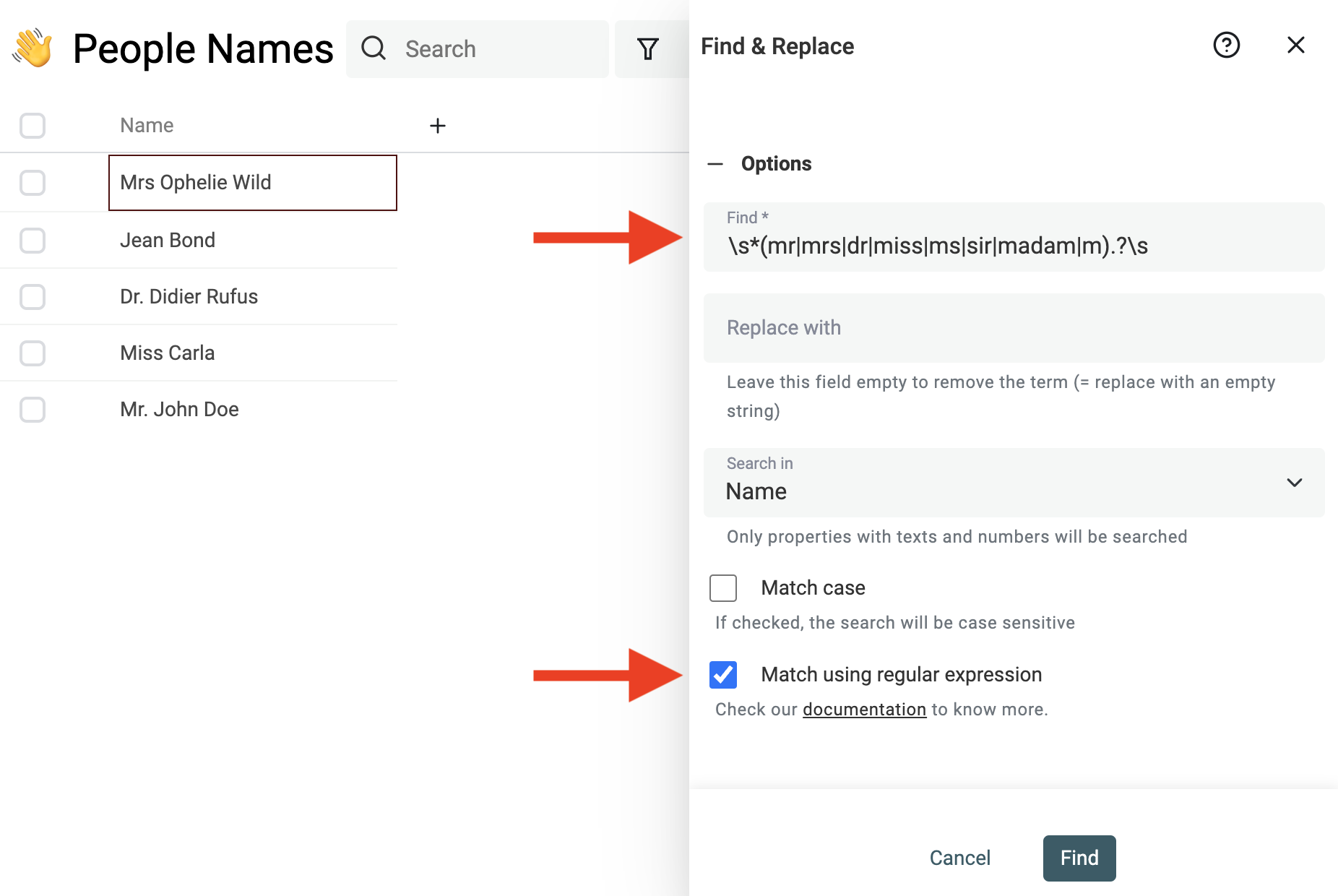The image comprises two screenshots of an address book or directory app. 

In the first screenshot, located on the left, you can see a waving emoji at the top left corner. To the right of the emoji, the text "People Names" is clearly displayed. Adjacent to this text, there's a search bar for easy navigation. Below this, a vertical list of five names is presented, each accompanied by an empty checkmark box on the right side. Notably, an arrow points from the second name, "Mrs. Ophelia Wilde," towards the second screenshot on the right.

The second screenshot features an "Options" tab at the top left. Directly beneath this tab is a text field labeled "Find," which includes options for various titles: Mr., Mrs., Dr., Miss, Ms., Sir, and Madam. Below this field, there's a "Replace with" section, which includes a searchable drop-down box labeled "Search in name." At the very bottom, there's a button labeled "Match using regular expression" next to a "Cancel" button located in the bottom right corner.